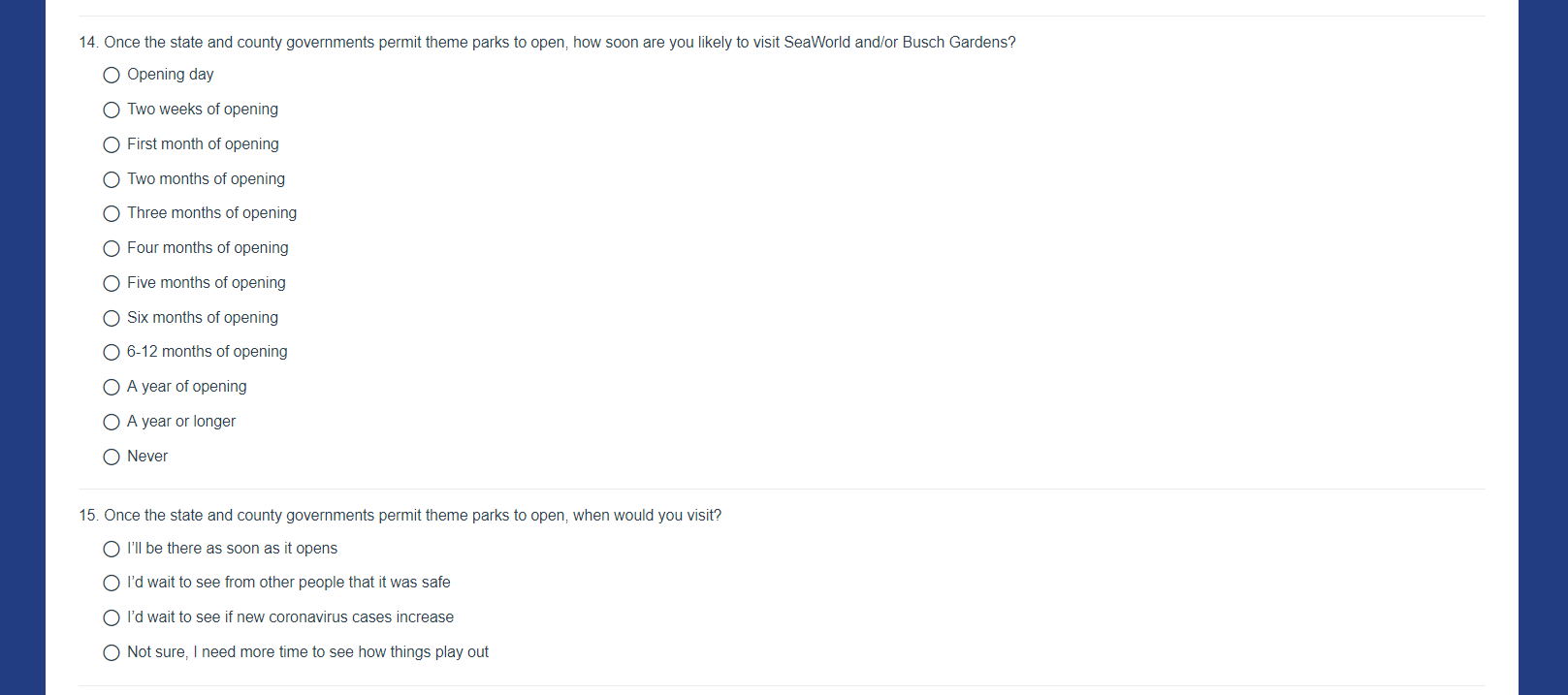This image captures a screenshot of a survey displayed on a webpage, framed with a blue border against a white background. The survey appears to be designed to gauge public sentiment about returning to theme parks following the easing of COVID-19 restrictions.

The first question, labeled as Question 14, reads, "Once the state and county governments permit theme parks to open, how soon are you likely to visit SeaWorld and/or Busch Gardens?" The question is followed by a series of options that range from immediate to indefinite timeframes: "Opening day," "Two weeks of opening," "First month of opening," "Two months," "Three months," "Four months," "Five months," "Six months," "Six to twelve months of opening," "A year of opening," "A year or longer," and an option for "Never."

The second question, labeled as Question 15, asks, "Once the state and county governments permit theme parks to open, when would you visit?" The provided response options are: "I'll be there as soon as it opens," "I'd wait to see from other people that it was safe," "I'd wait to see if the new coronavirus cases increase," and "Not sure. I need more time to see how things play out."

Both questions are written in black text, with a clear and organized layout that suggests it is directed at customers or a general audience to understand their willingness to return to theme parks in the aftermath of the COVID-19 pandemic. The structured format and presentation indicate that this is likely a screenshot taken from an online survey page.